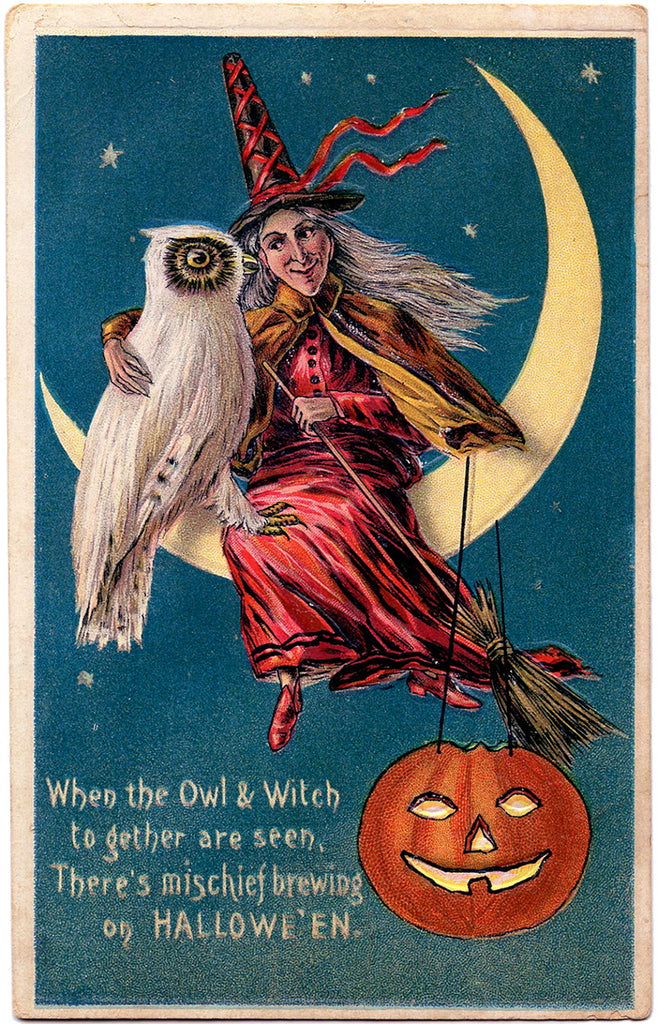This vertically aligned, portrait-style image resembles a vintage Halloween greeting card with a worn, beige border accented by brown. The central focus features a dark blue background adorned with delicate gold stars. Prominently, a large crescent moon occupies the upper half, upon which a smiling witch, dressed in a red dress and a black hat accented with red ribbon, sits alongside a white owl with a striking gold eye. The witch, who has long, straight gray hair, has her arm lovingly around the owl and clutches a broomstick. Suspended from the moon is a jack-o'-lantern, its face carved with triangular eyes and a ghoulish toothed grin, glowing in orange hues. In the lower left corner, white text reads: "When the owl and witch together are seen, there's mischief brewing on Halloween." This detailed illustration, likely intended as a holiday card or poster, exudes a nostalgic, old-world charm.